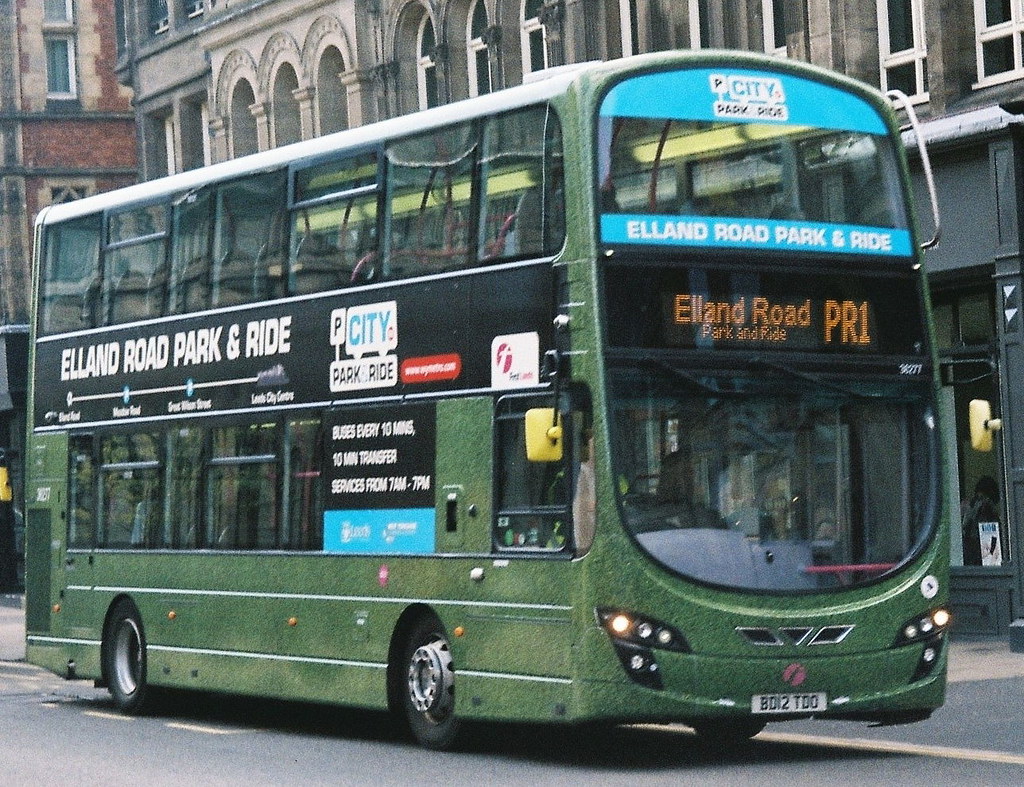The vibrant, full-color photograph captures a large, green double-decker bus driving on a nearly empty city road during the daytime. The historical architecture made of brick and stone in the background suggests the setting is in Europe. The bus, adorned with various advertisements, prominently displays the text "Elland Road Park and Ride" and "City Park and Ride." Notably, it offers a 10-minute transfer service running from 7 a.m. to 7 p.m., as indicated on both the side and digital front sign, which reads "Elland Road Park and Ride PR1." The absence of people and other vehicles emphasizes the focus on the bus and its role in public transportation. The overall image is clear and well-lit, despite some minor blurriness in the text on the side of the bus.